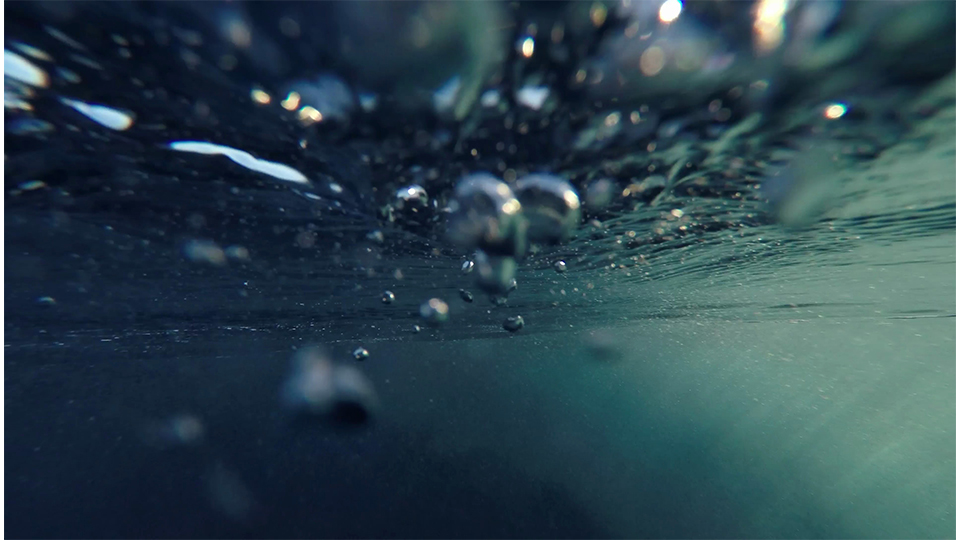The image depicts an underwater scene right below the surface, characterized by a bluish-gray hue with varying shades of dark and light. White lights and bubbles are scattered throughout, creating a dynamic and textured visual. Ripples on the water's surface can be seen in the distance, with light streaming in from one side. In the foreground, bubbles of various sizes, including large, silver orbs, float amidst dark and white areas. The bottom features a smooth bluish-gray area with hints of green, contributing to the overall depth and expanse, suggesting a deep and vast body of water like an ocean or a lake. The bubbles seem to be moving uniformly in one direction, as if influenced by an underwater current or an impact nearby, enhancing the sense of movement and life in the scene.